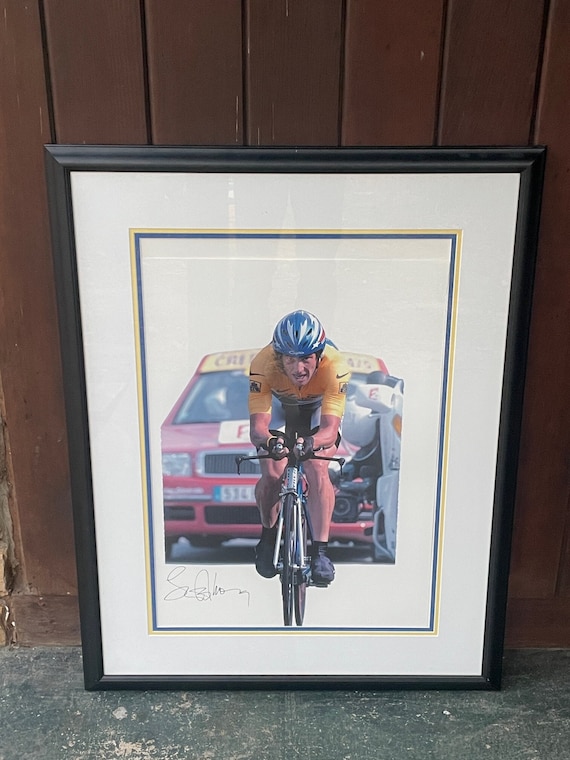This framed image, leaning against a dark oak wooden-paneled wall above a worn green floor, vividly captures a cyclist in the midst of intense action, possibly from the Tour de France. The cyclist, wearing a yellow Nike jersey and white bike shorts, pedals vigorously towards the camera while riding a black bicycle. He sports a blue helmet adorned with white flame-like stripes and wears black shoes. The determination is evident on his light-skinned face as his mouth is open, and he looks forward intently with dark hair peeking out. Following closely behind him is a red compact SUV or van, possibly serving as a pace or camera car, distinguishable by a slightly out-of-focus license plate and a yellow sign across the top. Also in the background, a white motorcycle is faintly visible. The photograph is signed in the bottom left corner, suggesting the possible involvement of the artist or photographer. The picture is bordered by a white mat with yellow and blue trim, all set within a sleek black frame, creating a striking contrast against the solid white background of the photo.